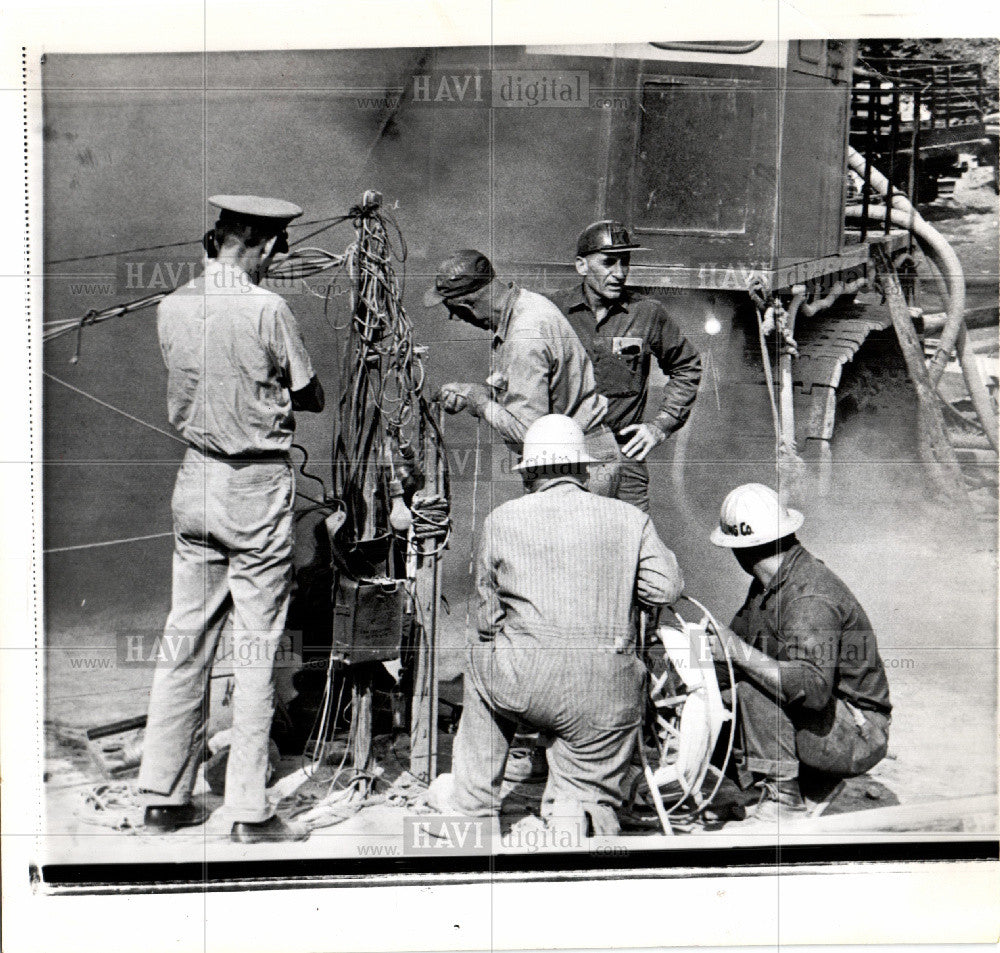This black-and-white photograph, possibly used for news or instructional purposes and marked repeatedly with the watermark "Havi Digital," features five men engaged in intense construction work. They are gathered around a complex vertical structure bristling with wires, which extends to approximately the height of the standing men before veering off to the left. The scene is dominated by a large tracked machine in the background, its interlocking wheel treads clearly visible, along with several large hoses extending from the machinery, one appearing dirty white. 

Three of the men are standing while two are kneeling near the base of the wire-laden pole, which might also suggest an electrical context. Three of the men sport hard hats, lending to the construction site's authenticity, while another wears a soft-sided baseball cap paired with glasses. The fifth man, dressed in what seems to be a uniform reminiscent of military or police attire, is distinguishable by his flat-topped cap and appears to be holding a phone receiver to his left ear, although his back largely obscures him from view. All individuals wear construction overalls, emphasizing their roles in this potentially urgent and intricate cleanup or construction task.